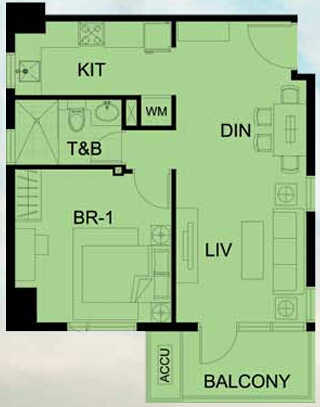This is a detailed, full-color blueprint of a home or apartment, presented in a green hue. In the top left corner, the layout indicates a kitchen area, labeled "KIT", complete with detailed illustrations of the sink and stovetop. Directly below the kitchen lies a region designated "T and B," shorthand for toilet and bath, featuring a shower area, a toilet, and a sink all clearly drawn in.

Adjacent to the bathroom, on the right, the blueprint marks an area labeled "WM," likely denoting a space for a washing machine. In the bottom left section of the plan, there is a bedroom labeled "BR1." This room is meticulously illustrated with a bed flanked by two nightstands, a rug, a dresser, and a window.

Moving to the right, a long, vertical, rectangular area is partially labeled "DIN," indicating the dining room. It features a dining table surrounded by four chairs. To the left of the dining area is the living room, marked "LIV." This space includes detailed drawings of a couch, a coffee table, a TV stand, and two small tables positioned on either side of the couch.

At the bottom of the layout, there is a small, vertical rectangular area labeled "ACCU." Finally, the area designated "balcony" completes the blueprint, illustrating an outdoor space accessible from the interior.